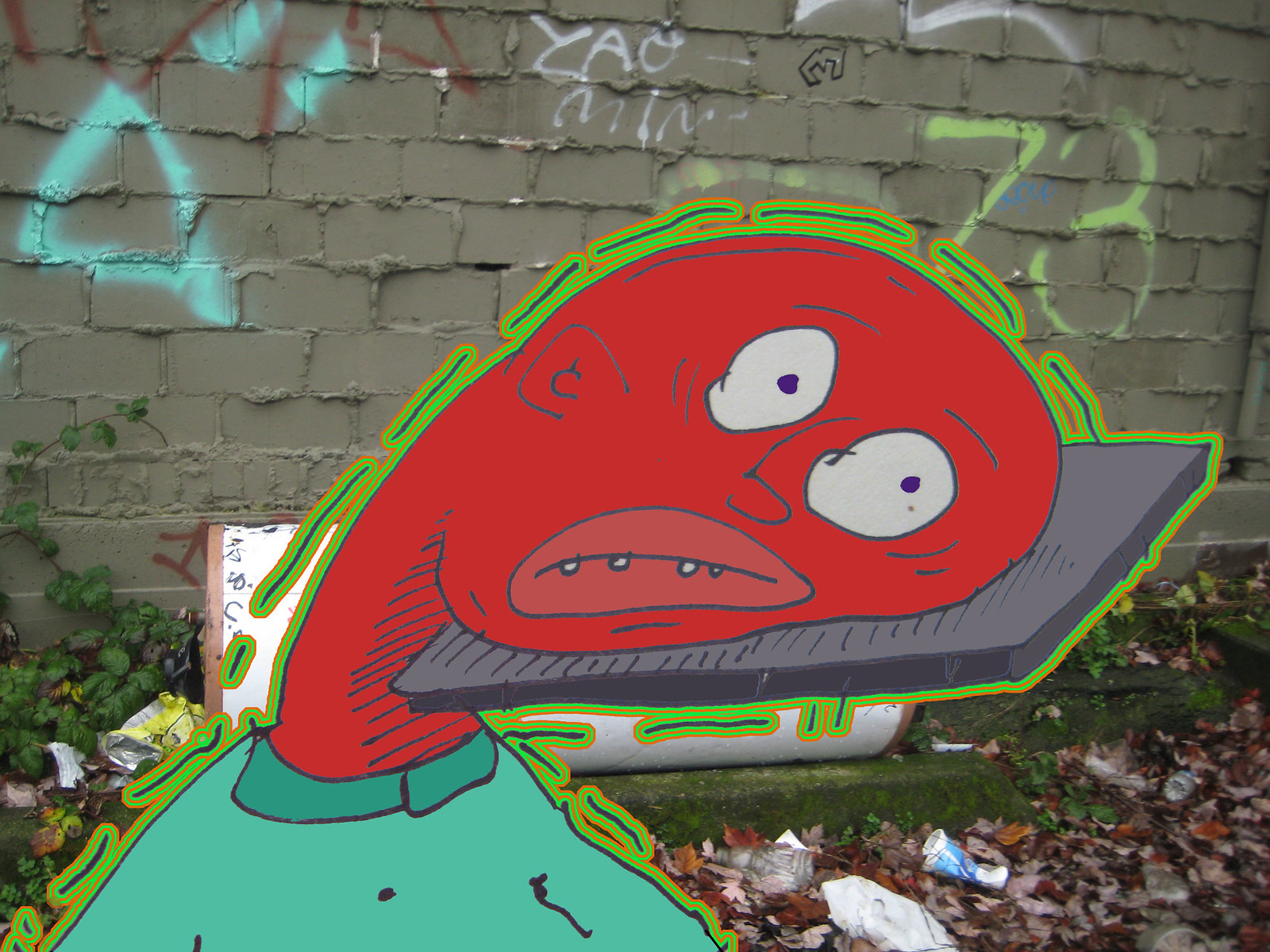The image combines a photograph and a computer drawing in a striking artistic piece. The background features a poorly constructed cinder block wall, uneven and slathered with excess mortar, adorned with various graffiti in multiple colors. Climbing ivy and weeds add a touch of green to a corner of the wall. Below, the ground is littered with dead leaves, smashed drink cups, fast food wrappers, chip bags, and other garbage.

Superimposed over this real-world chaos is a digitally drawn humanoid character with an oblong red face featuring a sideways mouth, four teeth, and disproportionately large eyes with small black dots as pupils. The character is dressed in a light green shirt with a dark green collar and has a dispirited expression. The red head appears almost squashed against a flat, rectangular gray object resembling a stone slab or a book. Surrounding the character is a psychedelic outline in green, orange, and blue hues, adding to the surreal atmosphere of the composition.